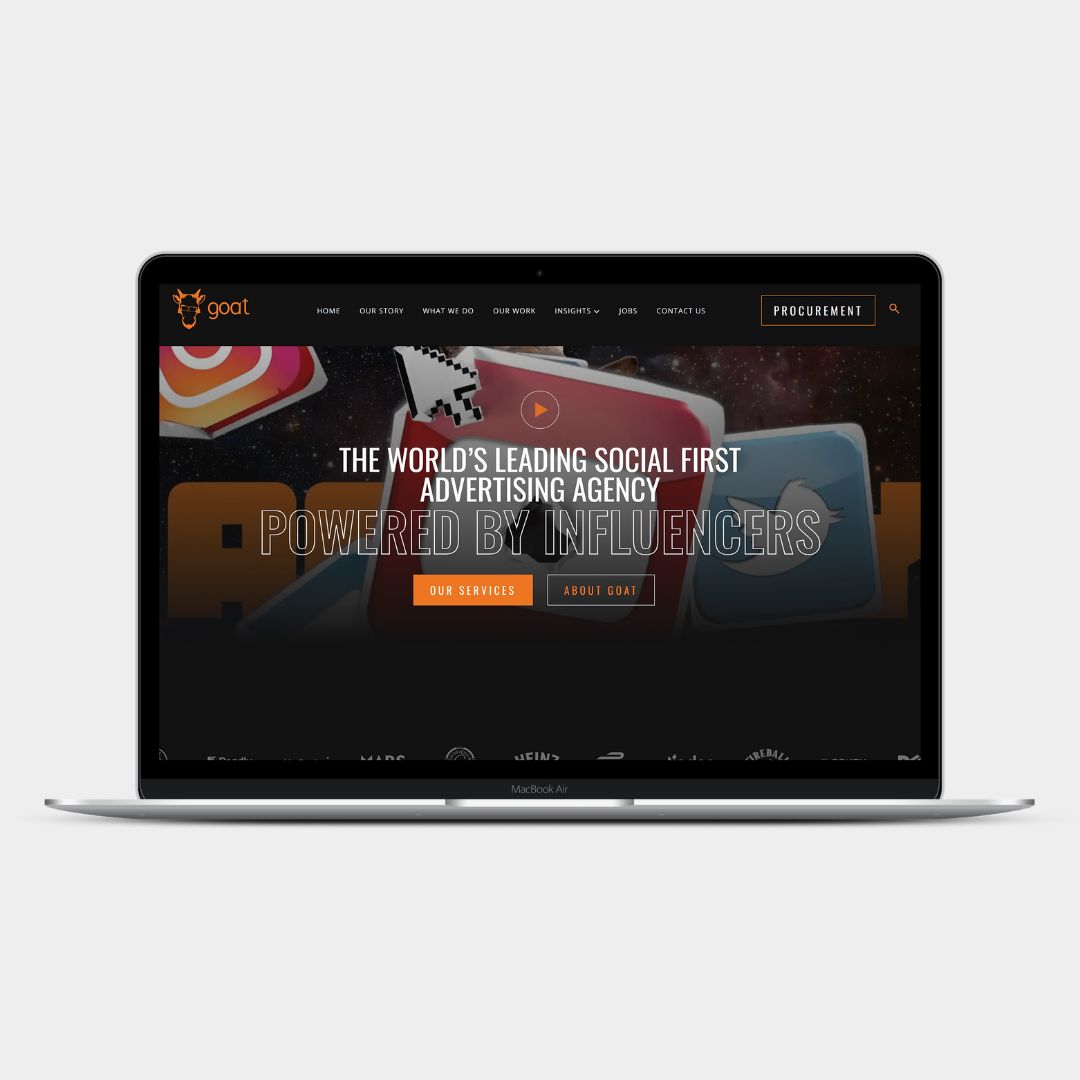The image depicts a photograph of a MacBook Air placed on a light gray background. On the MacBook Air's screen, a website is displayed. The website features a top navigation bar on a mostly black background with orange lettering. On the left side of this bar, there's a logo that might read "Goat" or "Goal." The navigation options listed are: Home, Quick, What We Do, Our Work, Insights, Jobs, and Contact Us. On the right side of the navigation bar, there is a prominent "Procurement" button and a magnifying glass icon for search functionality.

Below the navigation bar, the main portion of the screen displays a bold statement in white outlined font: "The world's leading social-first advertising agency powered by influencers." Below this statement, there are two Call-to-Action buttons. The one on the left has an orange background with white text that reads "Our Services." The button on the right has a black background with orange text that reads "About Goal" or "About Goat."